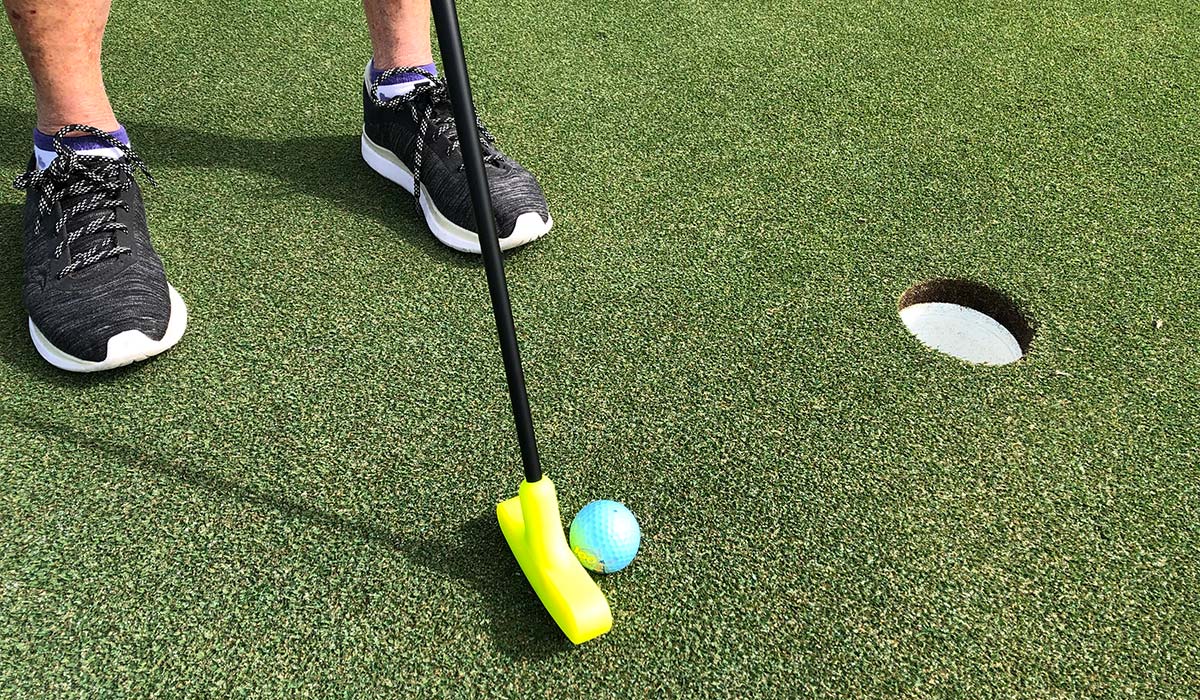The image shows a close-up scene of a miniature golf setup, focusing on the lower legs and feet of a golfer. The golfer, whose light-skinned legs are visible above their low socks, is wearing black athletic shoes with white soles. The artificial green turf, giving an appearance of grass, covers the ground. Central to the frame is a blue golf ball positioned right in front of a plastic black golf club with a neon yellow head. The ball and club are poised for a putt towards a small, circular hole on the right side of the frame. The hole is fitted with a white plastic cup to catch the ball. The positioning and detail suggest this is a practice area, possibly indoors.